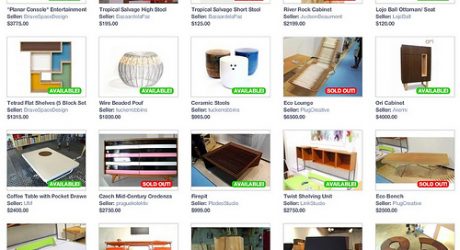This screenshot captures a portion of a website displaying various products against a white background. Each product is presented in uniform, slightly-rounded, thin, light gray-outlined frames. The product images within these frames feature a status tag in the bottom right corner; these tags are either green with white text reading "Available" or red with white text reading "Sold Out!" 

Each product listing is formatted with a bolded product title in black text beneath the image. Below this title, left-justified alongside the frame’s border, is the word "Seller" in bold text, followed by the seller's name in lighter gray text to the right. Further down, also left-justified, is a bolded price prefixed by a dollar sign.

The first product listed is "Tetrad Flat Shelves (Five Block Set)" sold by an unreadable individual due to blurriness, priced at $1,215.00. The accompanying photo depicts an abstract wooden shelving set designed to resemble a game of Tetris. 

All other products on the website follow a similar layout and presentation format.